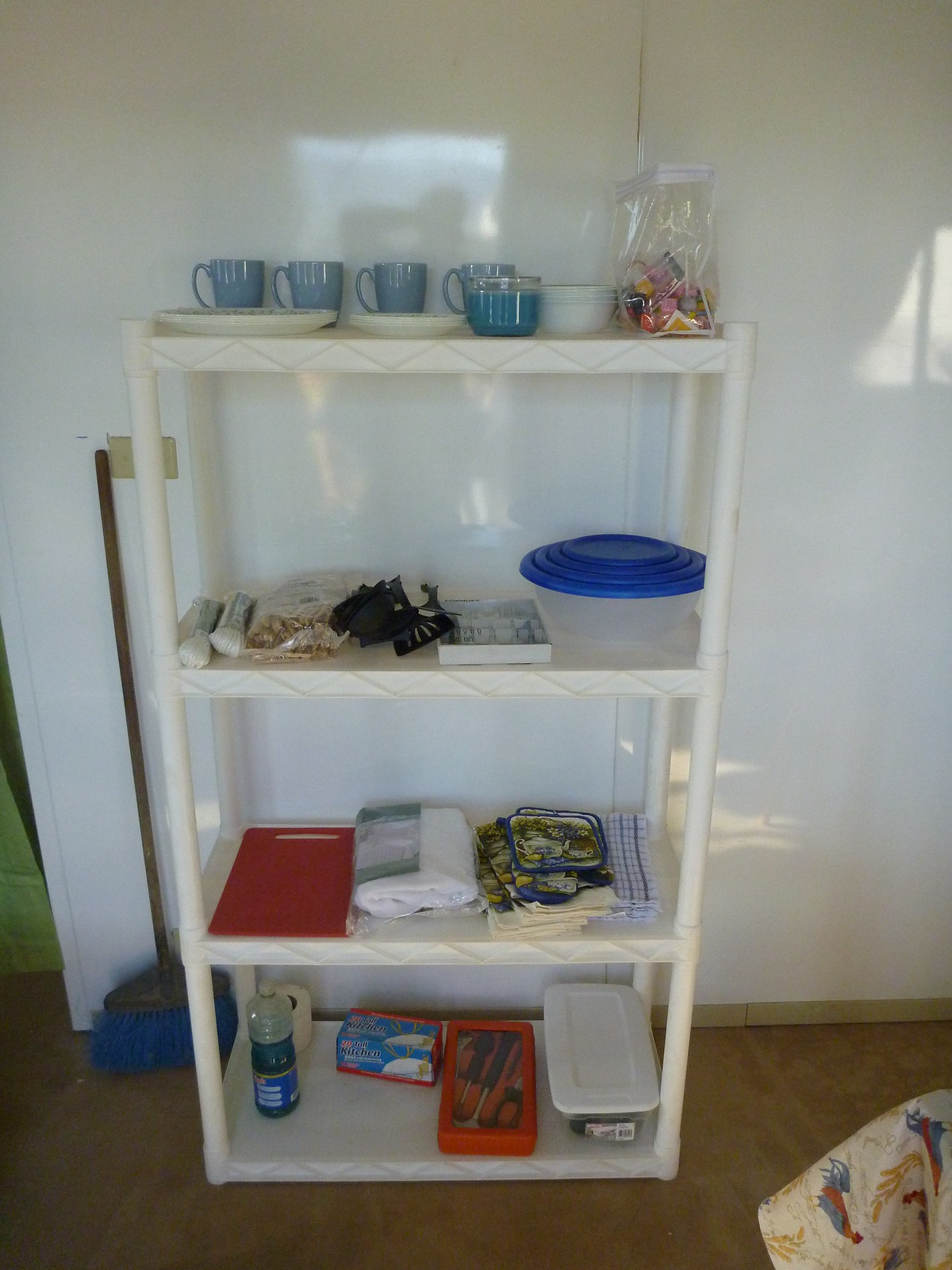A color snapshot taken inside a home captures the interior's simplicity with a focus on a white wall. The wall, devoid of any decorations or features, stands as the primary subject. However, its surface is animated by the interplay of light and shadow. These reflections, likely cast from a door or window on the room's opposite side, create a dynamic pattern, adding depth and interest to the otherwise mundane scene. The light, filtering through, forms soft, diffused shapes, hinting at the presence of unseen elements beyond the frame and giving life to the static image.